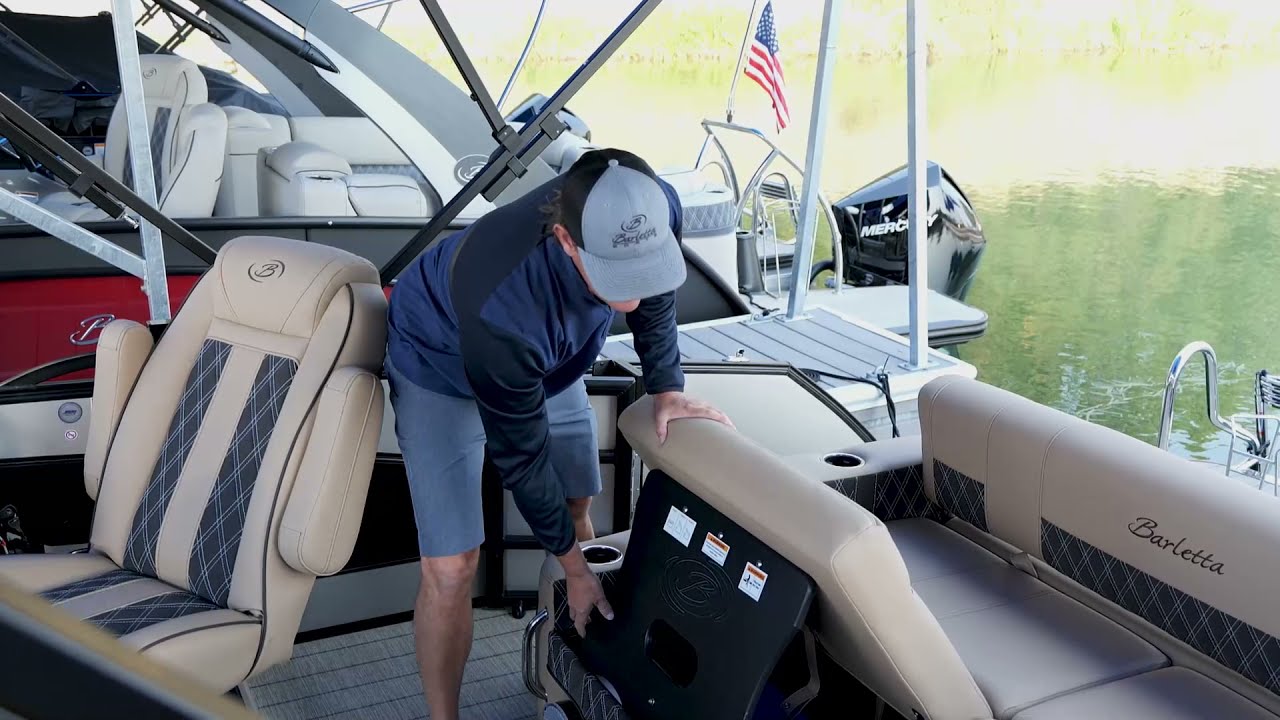In this photograph taken from inside a motorboat named Barletta, a man is the central focus, positioned in the middle of the boat. He is bent over, obscuring his face, and is wearing a gray cap with black text, a blue long sleeve shirt or jacket, and blue or possibly gray shorts. He appears to be adjusting or lifting a black square object with a hole in its center behind a cream-colored seat. This seat, along with another on his left, is cream-colored with the Barletta logo in a navy blue with white cross-hatching design. To his left, there is a tan captain’s chair with a raised back featuring navy blue stripes with white hatching down the middle. The boat has beige and navy blue fabric, contributing to a cohesive color scheme.

In the background, the American flag is visible, fluttering above the back of the boat. Beyond this, another boat is docked, primarily gray with white seats and a red stripe, partially visible. The motor, which reads Mercury, is discernible at the back of the second boat. The water surrounding these boats exhibits varying shades of green and yellow, reflecting the sunlight.